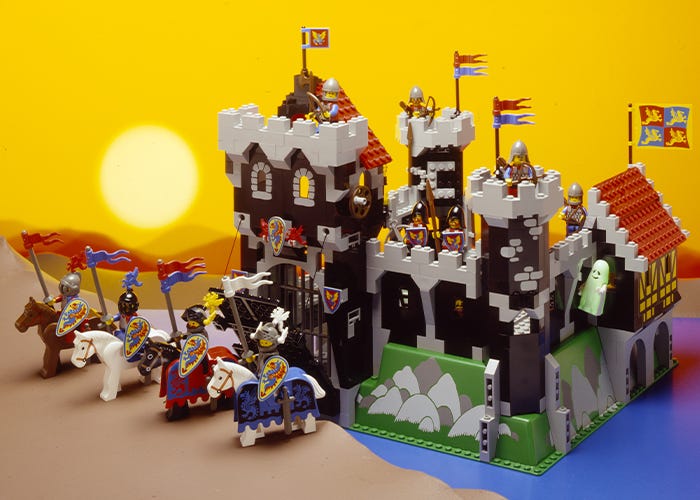The image is a detailed, horizontally-oriented photo of an elaborate Lego castle set. The castle features multiple turrets—the largest being brown with a white top and a bit of red roof, while the others are primarily gray. There is a smaller house in the back with wood sides and a red roof. The green-painted front wall has illustrations of boulders. The castle's facade includes a black structure with grey accents, shields, and red dragon crests above a partially lowered drawbridge. The entire scene is set against a beautiful yellow sunset sky, adding warmth to the outdoor pretend setting.

In front, four or five Lego knights are mounted on horses, three white and two brown, each knight carrying a flag and their horses adorned with long drapings. The castle appears to be situated in a sandy area with a moat-like water depiction surrounding it. Several Lego figurines are positioned inside and atop the castle towers, adding to the lively scene. Additionally, a green ghost figure can be seen on the right side of the image. Overall, the photo captures a vibrant and creative Lego setup, intricately assembled as if imagined by a skilled child.